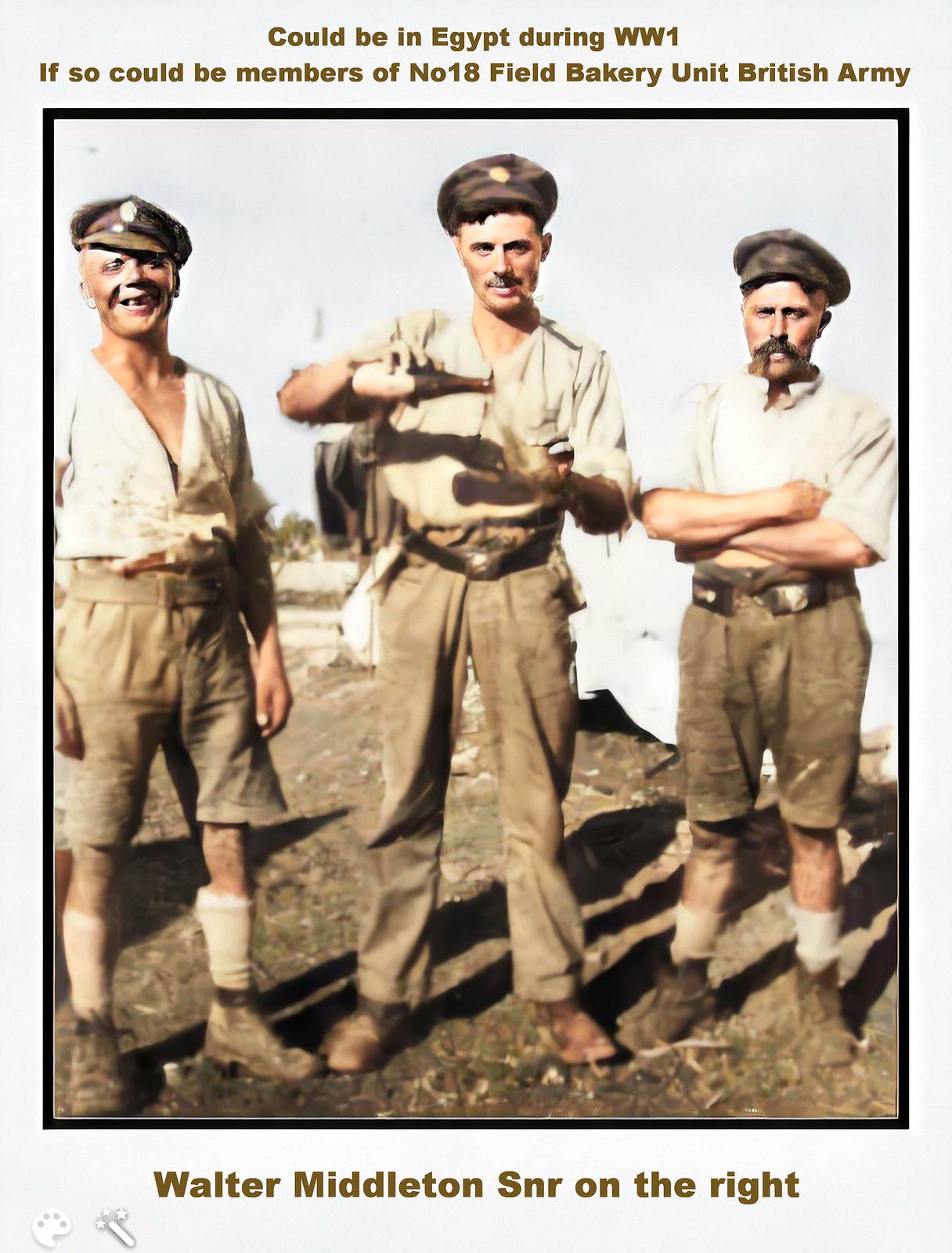This color photograph, potentially from World War I, depicts three young men standing on a dirt surface and possibly belonging to the No. 18 Field Bakery Unit of the British Army, perhaps stationed in Egypt. They are all dressed in military garb consisting of light tan shirts and dark brown trousers. The men on the left and right are wearing shorts, long socks, and boots, whereas the man in the center is dressed in long pants and boots. Each man is sporting a similar military cap. The central figure, with a mustache and a cigarette dangling from his mouth, is seen pouring a beverage, likely beer, from a bottle into a glass. The man on the left, smiling broadly and missing a few teeth, adds a touch of levity to the scene. The man on the right, identified as Walter Middleton Sr., also has a mustache and is seen with a pipe in his mouth. Behind them is a white structure, possibly a tent, contributing to the war-time setting of the image.